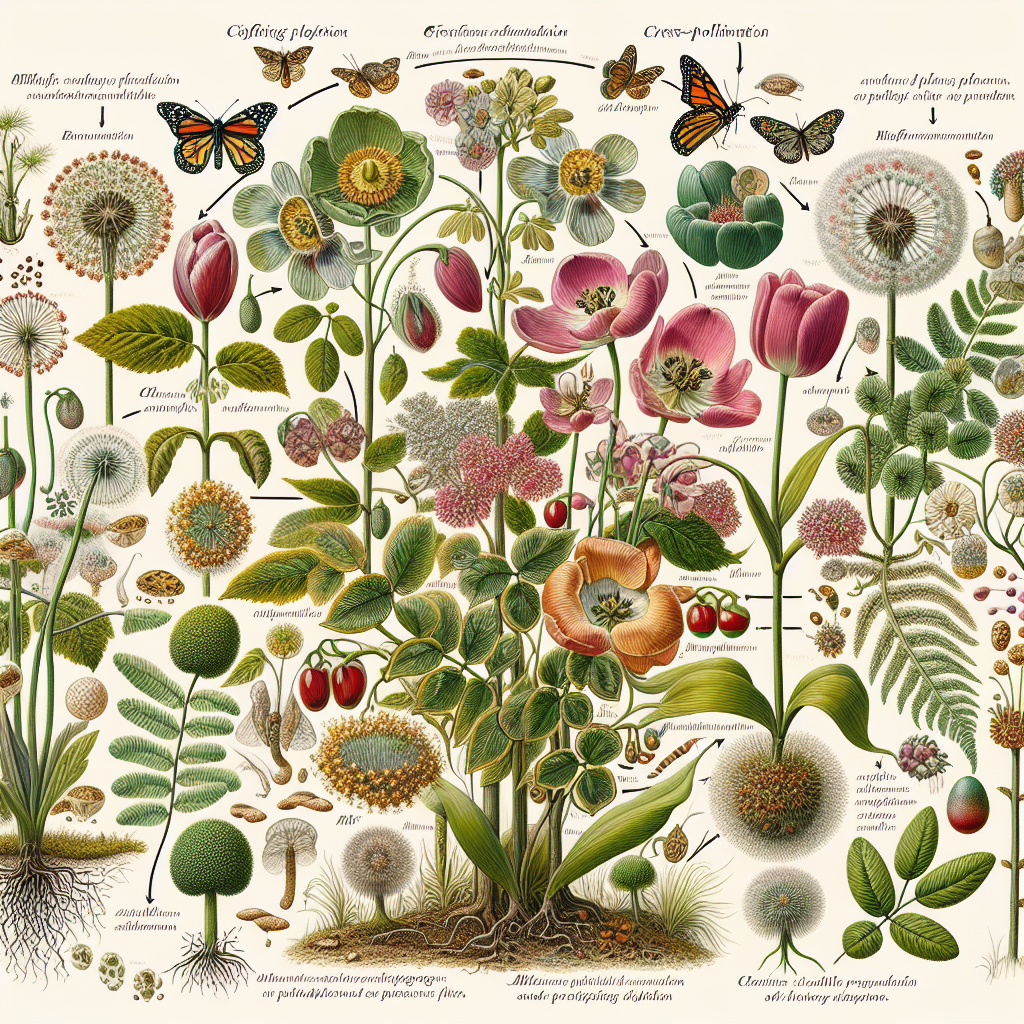The illustration depicts a detailed and vibrant scene of various butterflies and flowers set against an off-cream background. Monarch butterflies, notable for their striking orange and black wings adorned with white speckles, dominate the composition, along with a few smaller, off-white and beige moths. The drawing exquisitely captures the pollination process, with butterflies interacting with numerous flowers, including tulips, poppies, and dandelions. Some flowers are fully bloomed, while others are not. Central to the image is a prominent green plant with visible roots extending into the soil at the bottom, surrounded by a variety of other plants and vines. The scene is further enriched with cursive text that diagrams and describes the botanical and entomological details, enhancing the educational essence of the artwork. The colors span a diverse palette, from deep pinks and dark greens to yellows and light greens, combining to create a richly detailed and scientifically informative illustration.